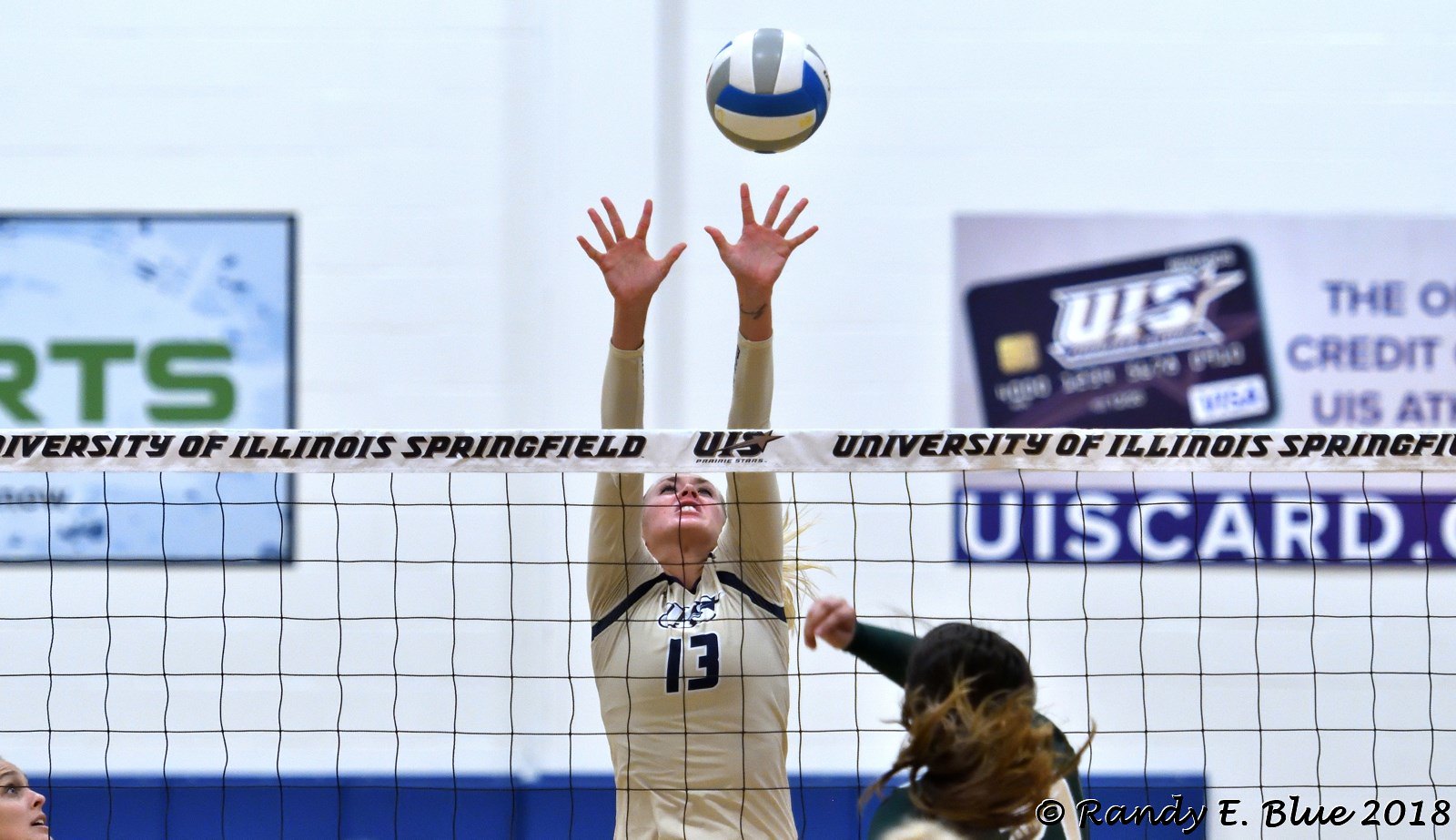The photograph captures an intense moment in a college-level women's volleyball game, set in an indoor gymnasium adorned with sponsorship logos. Central to the image, a player from the University of Illinois Springfield, identifiable by her number 13 (in navy font), is about to spike the ball over the black net, which proudly displays "University of Illinois Springfield" at its top. This athlete, a Caucasian woman with long blonde hair, is captured mid-action: arms fully extended, fingers spread, reaching for a volleyball that is suspended near the top of the image. The volleyball itself is multi-colored with stripes in blue, white, yellow, and grey. On the opposing side, one can make out another player, a brunette with some blonde highlights, poised to block the spike, though her face is partially obscured. Additional details include a watermark on the bottom right corner reading "Randy E. Blue, 2018," and the presence of a partial face of another brunette player in the bottom left corner. The gymnasium walls, painted a very light blue, feature commercial advertising such as a green "RTS" logo and a purple UIS Visa card ad, adding context to the vibrant athletic scene.